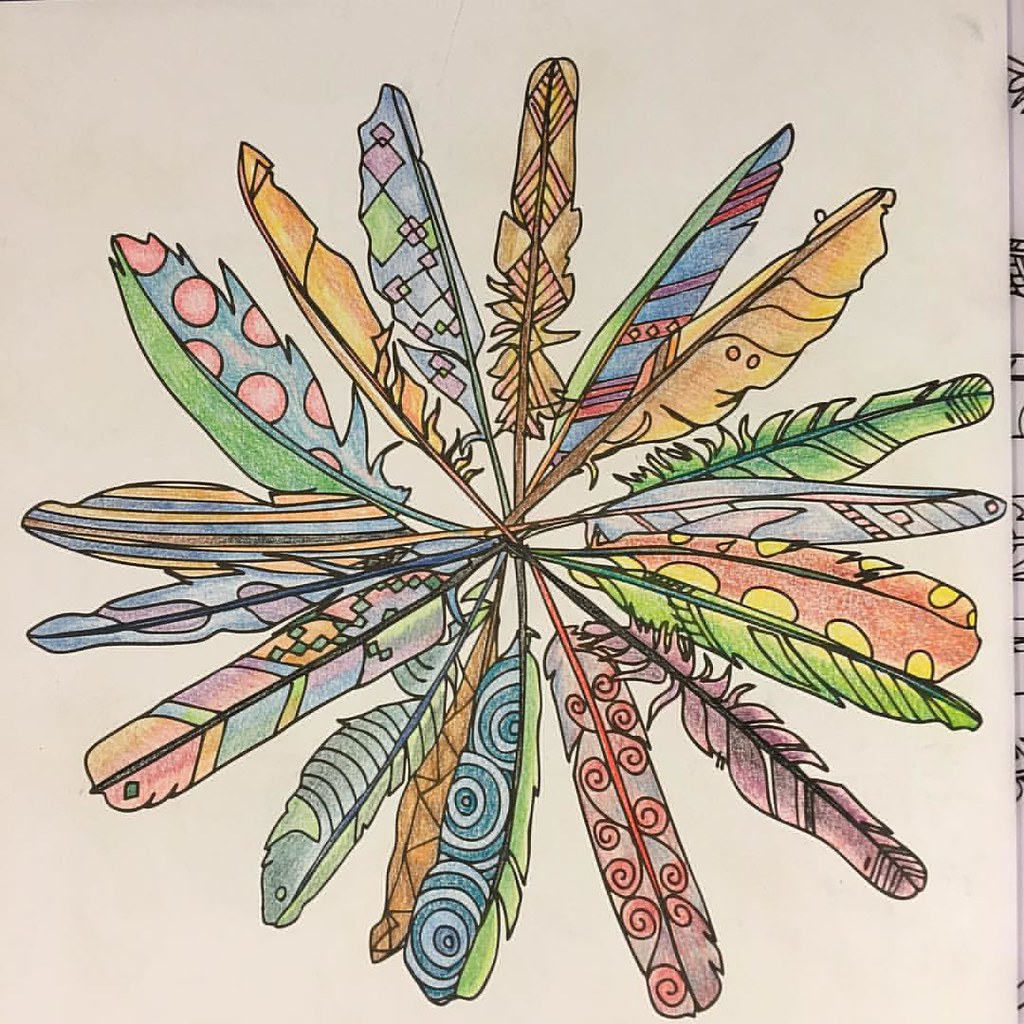The image depicts a vibrant and intricate arrangement of hand-drawn feathers, radiating in a circular pattern on a sheet of construction paper. Approximately 20 feathers converge at their bases and extend outward, resembling a starburst. Each feather is meticulously illustrated, showcasing an array of vivid colors including shades of pink, blue, and various other hues, creating a visually rich and dynamic artwork. The feathers are not real; they are drawn with precise detail, contributing to the overall visual harmony of the piece. This thoughtful and colorful design captures the essence of artistic creativity and expression.